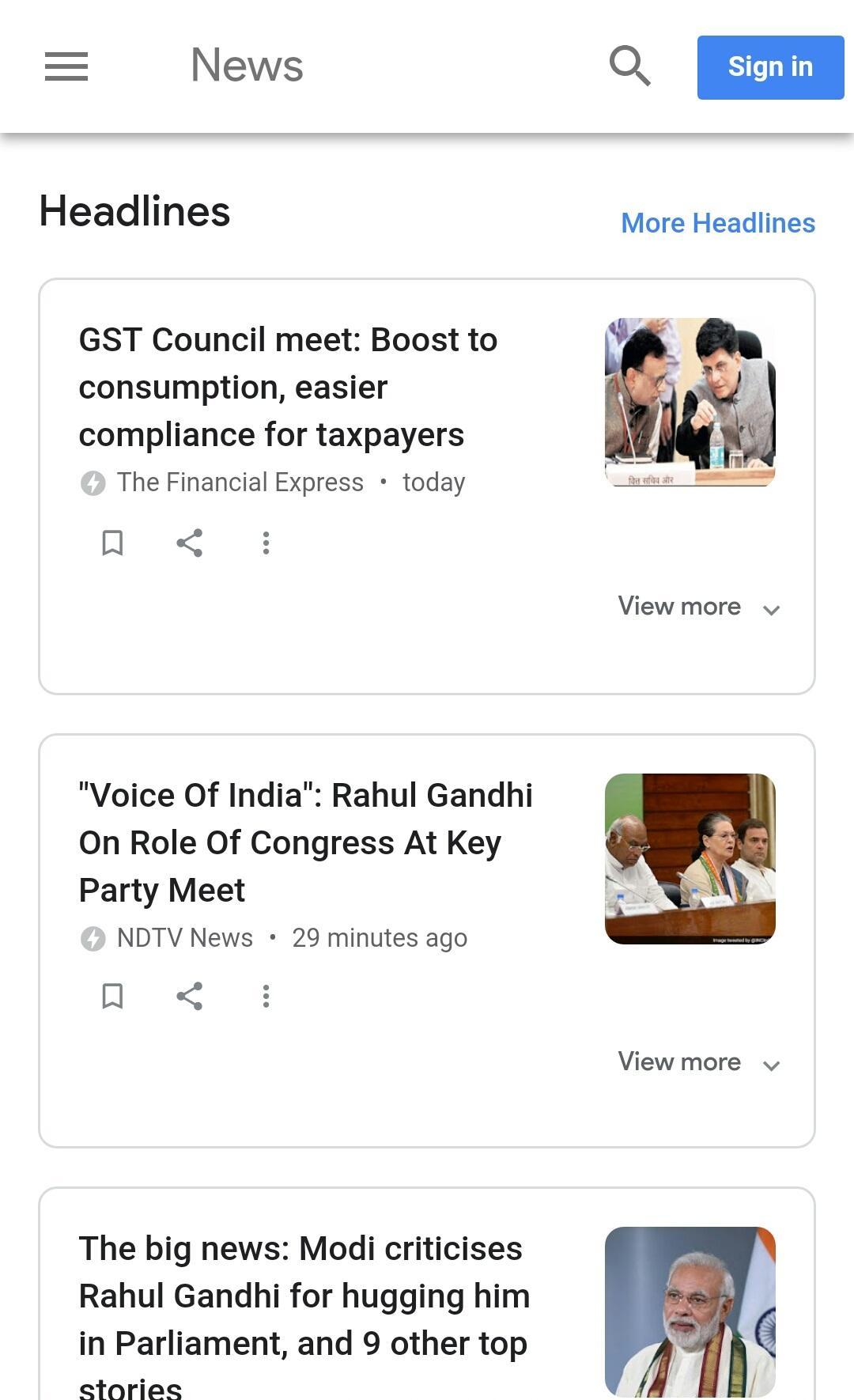The image displays a user interface of a news website with a white background and black text, featuring a collection of headlines focusing on Indian politics. At the upper left corner, there is a "News Headlines" title accompanied by a menu icon with three horizontal bars, likely for navigation. On the upper right, a user can find a "Sign In" button and a magnifying glass icon indicating the search function.

Prominently featured are three main headlines: 
1. "GSC Council Meet Boosts the Consumption, Easier Compliance for Taxpayers"
2. "Voice of India: Rahul Gandhi on Role of Congress at Key Party Meet"
3. "The Big News: Modi Criticizes Rahul Gandhi for Hugging Him in Parliament, and Nine Other Top Stories"

These headlines highlight relevant political events and controversies. The articles are from different news outlets and appear to have been published around the same time. To the far right of the page, there is a "More Headlines" button for additional news stories. Each article includes options to save or share it via various platforms.